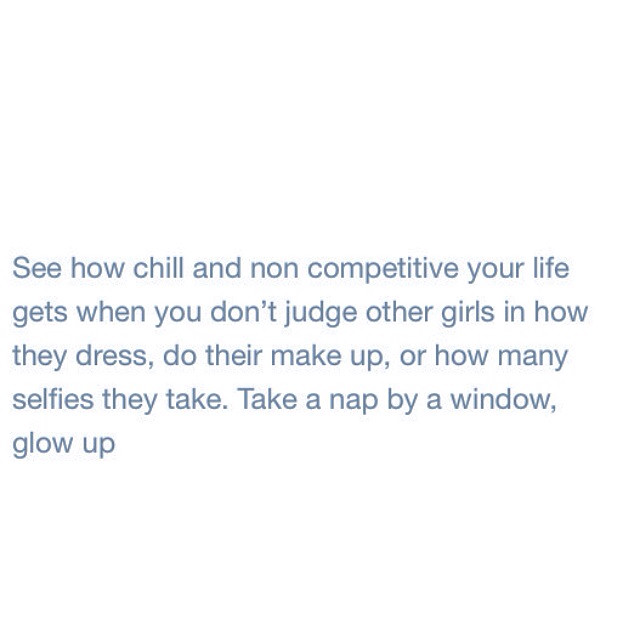The image features a minimalist design with a solid white background and a block of left-aligned text, centered vertically with ample blank space around it. The text is written in a light grayish-blue sans serif font and extends over five lines, sharing an inspirational message. It reads: “See how chill and non-competitive your life gets when you don't judge other girls and how they dress, do their makeup, or how many selfies they take. Take a nap by a window, glow up.” The phrase "glow up" is placed on the last line, subtly emphasizing its importance. The absence of a period at the end of the text adds to its casual, conversational tone. The overall style evokes a motivational social media post aimed at promoting kindness and self-care.